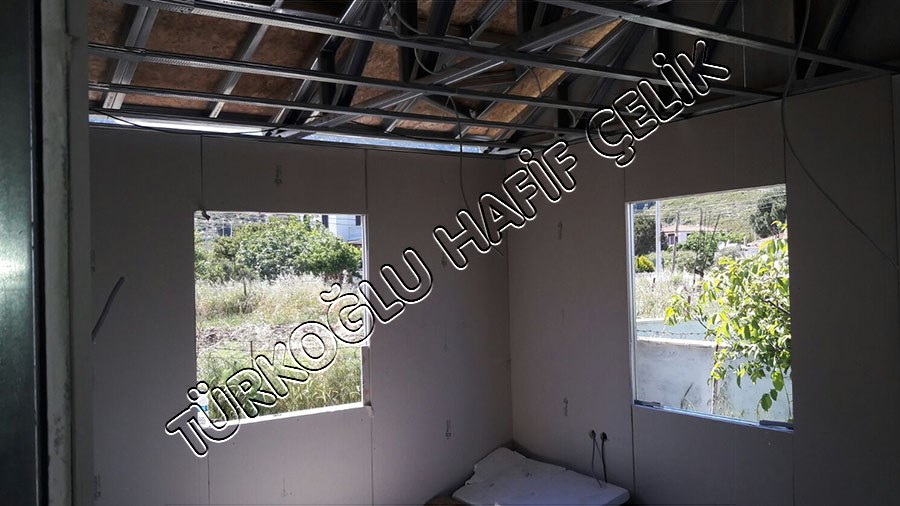The full-color photograph captures an indoor scene of a room bathed in daylight, suggesting it’s undergoing renovation. The space is stripped down to its essentials, with bare, possibly drywall, walls showing signs of wear and tear. The ceiling is unfinished, exposing wooden rafters and roof decking. Two windows are visible; one on the right side of the room reveals a sunny outdoor view with a tree and a white structure that might be a swimming pool, while the other window offers a glimpse of grass, a bush, and additional foliage.

Inside, an indistinct white object rests in the corner of the room's floor, and some wires protrude from the walls, indicating ongoing construction. The light inside the room is dim, casting shadows on the walls. In the background of the exterior view, a low white wall, more grassy areas, trees, and a few distant houses can be seen, suggesting a residential environment.

Stretching horizontally across the image is a watermark, reading "Turkoglu Hafif Çelik," possibly indicating the name of the company involved in the renovation project. The letters appear in a clear, somewhat transparent font, subtly blending into the photograph’s context.